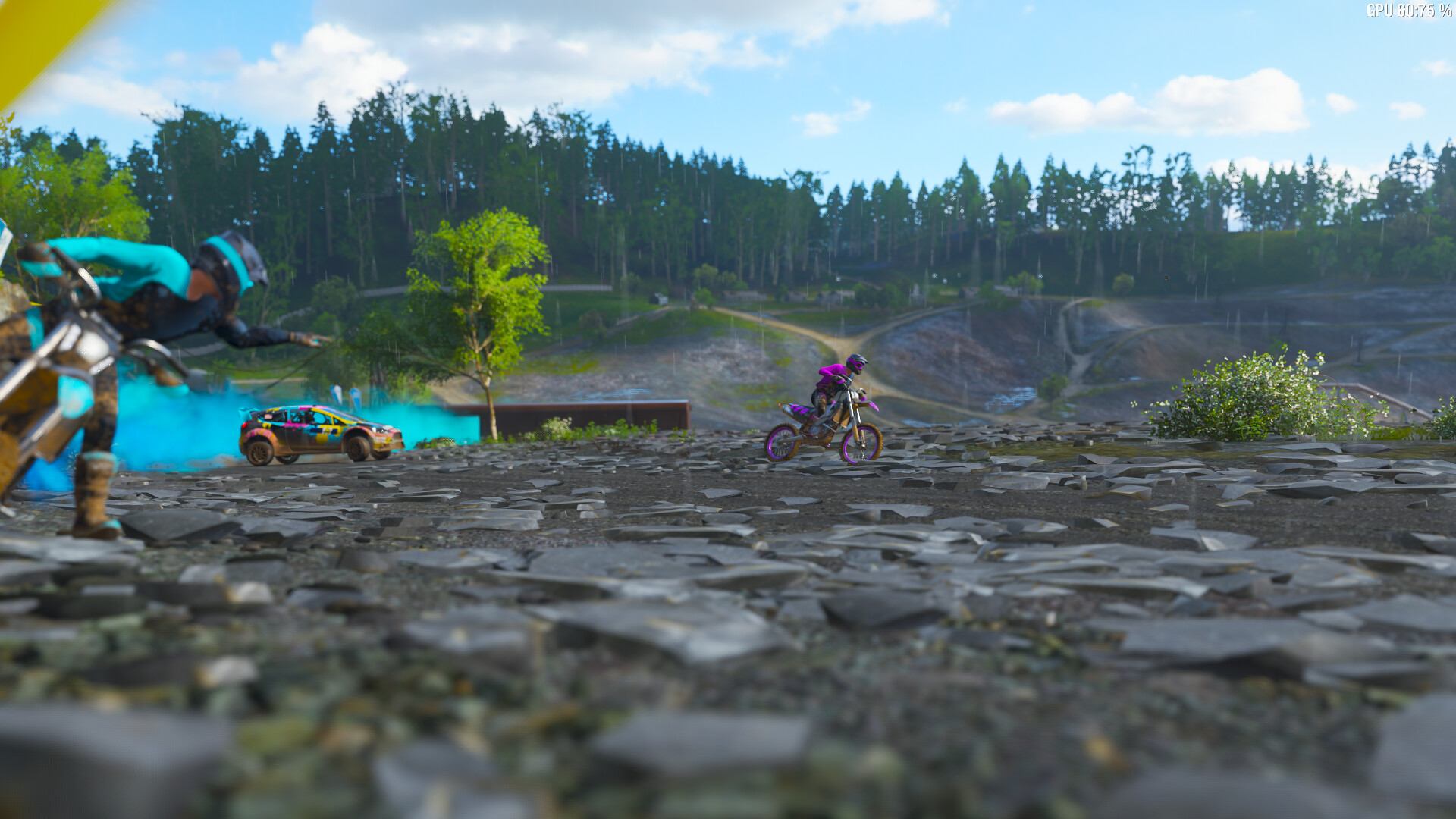In this computer-generated image captured at ground level, the scene is set on a rocky terrain composed of flat stones. In the background, there's a gently sloping hill with a discernible trail, bordered by patches of grass. The landscape is dotted with lush green trees, under a clear blue sky with minimal cloud cover. 

Prominent in the foreground, there are two men on motorbikes. The man positioned centrally in the photo, slightly further back, is attired in a purple outfit and riding a matching purple bike. To the left, another man wears a black and teal outfit; however, only the handlebars and front fork of his bike are visible, and his leg appears to be cut off from the view. Further back, part of a car is also visible, though it seems disproportionately small compared to the men and bikes, occupying about half their size in the image.